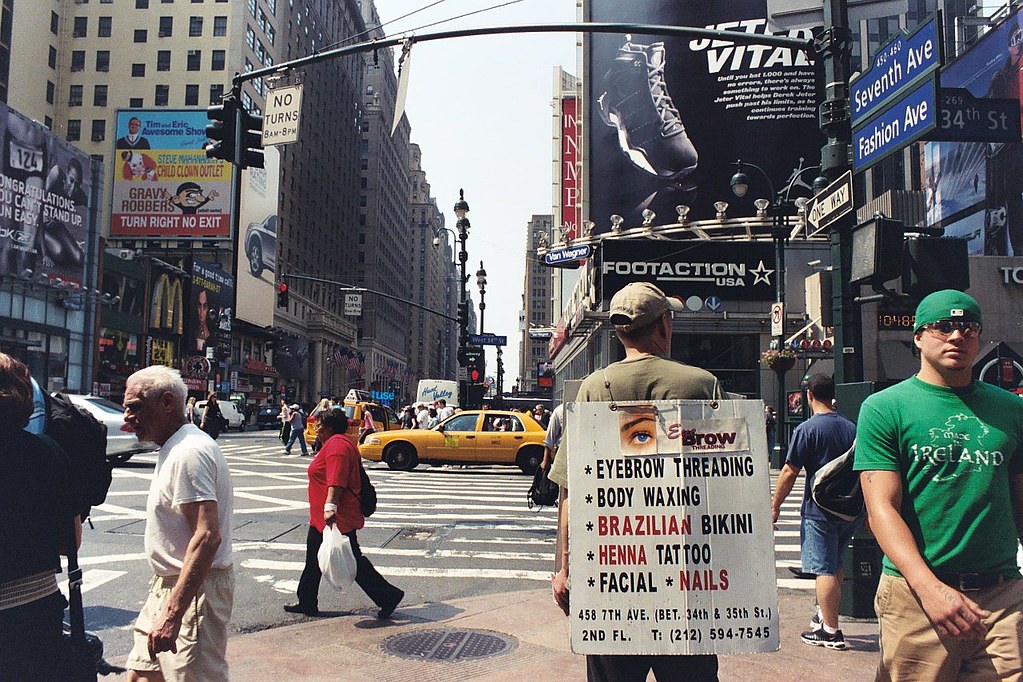This bustling city street scene, likely in New York City, captures the vibrant urban life with numerous pedestrians and yellow cabs crossing a busy intersection. On the left, tall buildings rise, some reaching 15 to 20 stories high, with a visible McDonald's on one of the lower levels. The right side of the photo features a man walking towards the camera, dressed in a green cap, green 'Ireland' t-shirt, and khaki pants. Next to him, in the center, a man wearing a brown cap and shirt carries an advertising board listing services like eyebrow threading, body waxing, Brazilian bikini, henna tattoos, facials, and nails, along with the address 458 73rd Avenue, between 14th and 15th Street.

Above this man is a large Foot Action USA sign, prominently featuring a black sneaker and the name "Vital" in the upper right corner of the sign, with "Jeter Vital" written underneath. In the far right upper corner, a blue street sign reads "7th Avenue, Fashion Avenue," beneath which a one-way sign points away. The photo's upper section shows a streetlight over the road, adorned with a white "No Turns" sign.

To the left side of the image, a woman in a red shirt steps off the sidewalk, clutching a white bag, and nearby an older man in a white shirt and tan shorts walks. The diverse array of advertisements and storefronts, including a notable McDonald's, captures the essence of a lively downtown area teeming with activity and commercial variety.